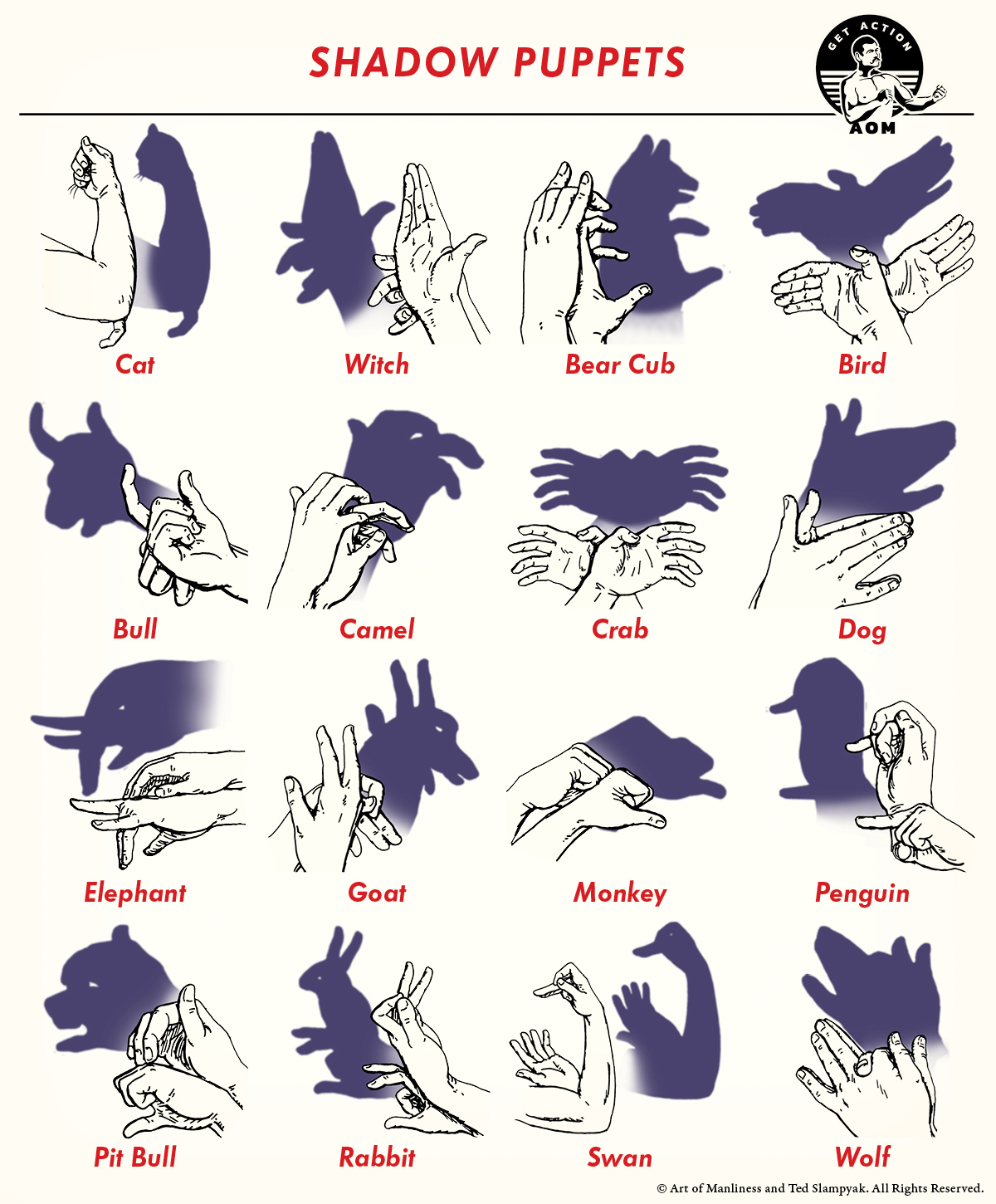The image is a detailed, hand-drawn diagram demonstrating how to create various shadow puppets using your hands and arms. Titled "Shadow Puppets" in red text at the top, the instructions are arranged in a 4x4 grid on a white background, each box showcasing a different shadow puppet. Each illustration depicts hands in a specific position to form the shadow of an object or animal, with a corresponding black shadow displayed behind the hands. The shadows include a cat, witch, bear cub, bird, bull, camel, crab, dog, elephant, goat, monkey, penguin, pit bull, rabbit, swan, and wolf. Each shadow puppet is labeled in red text underneath the shadow image. To the upper right of the title, there is a logo of an old-school boxer with the letters "A-O-M" beneath him. Additionally, small, unreadable text and a copyright notice are present in the bottom corners of the image.